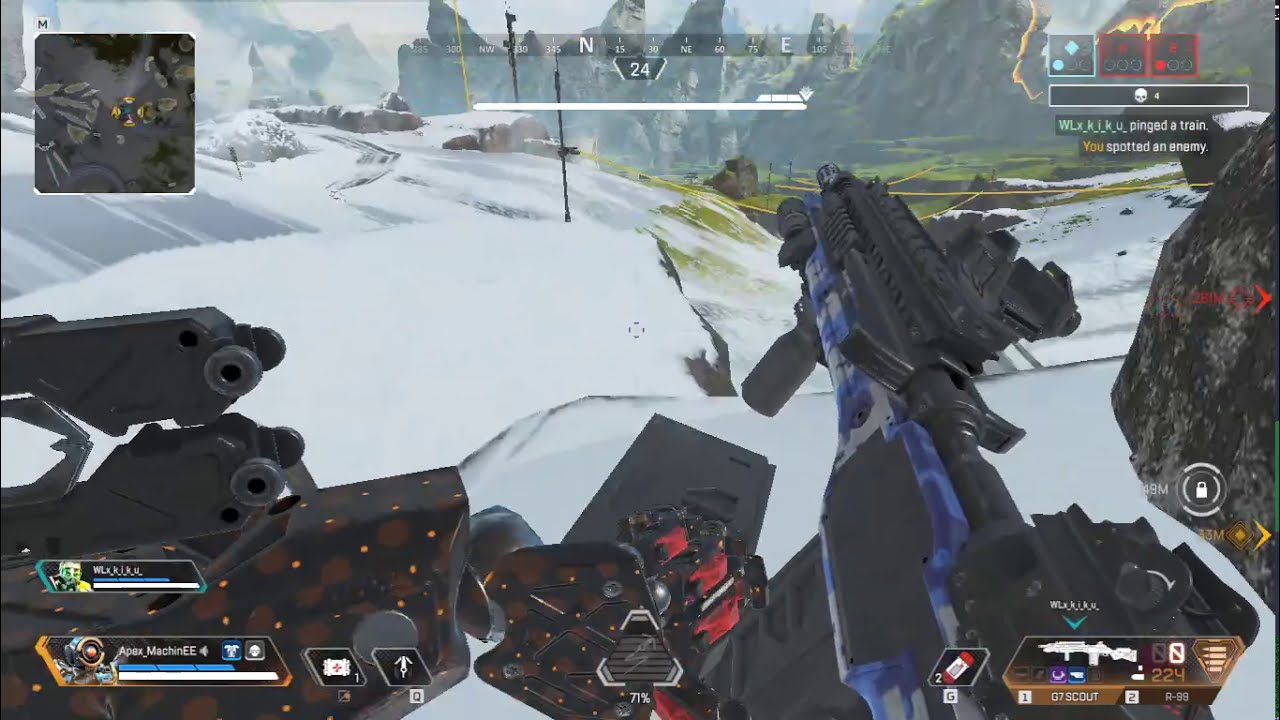This image is a screen capture from a first-person shooter video game, depicting a slightly pixelated, snowy landscape in the foreground with jagged rocks and snow-covered terrain. In the background, towering mountains with hints of greenery can be seen. The player's view includes a detailed interface: a mini-map in the top left corner, which indicates a spotted enemy, and a health bar for characters at the bottom left. The weapon selection is visible in the bottom right corner, currently showing a bluish-black rifle with white and gray camo accents, held by the player's character, whose gloved, possibly robotic, hands are visible. The gloves appear black with orange and red highlights. Additional HUD elements include a compass at the top center indicating cardinal directions with degrees of latitude, and an open chat box in the top right corner, creating an immersive and strategic gameplay environment.